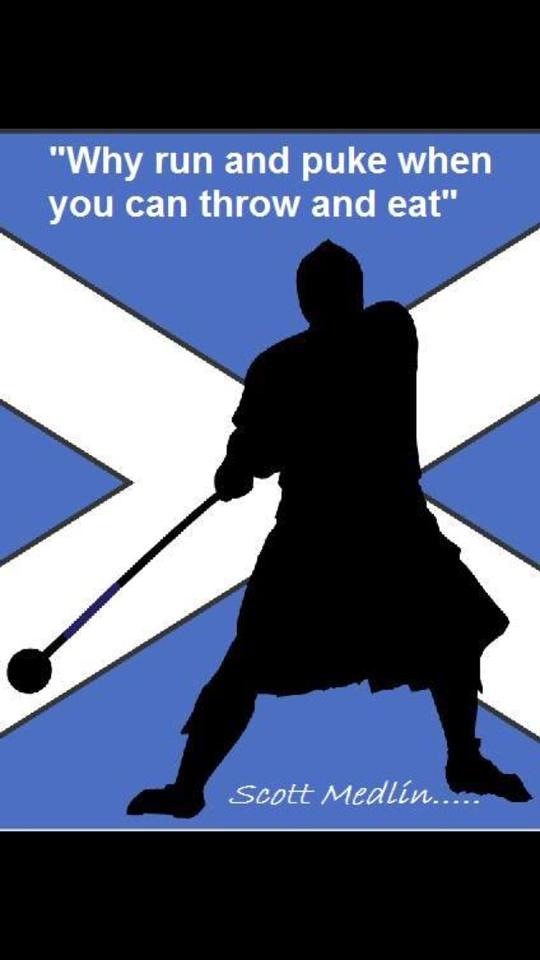The image resembles a meme or an online creation featuring distinct black bars at the top and bottom. Central to the image is a design reminiscent of the Scottish flag, distinguished by its blue background and white X cross. Superimposed on this background is a black silhouette of a man, potentially wearing a kilt and appearing to be in the act of throwing a weight. This silhouette, possibly also wearing a pointed helmet or having styled hair, adds a medieval, Highland warrior-like vibe to the composition. The figure is bracing and positioning his feet for stability while holding a long stick with a circular end, suggesting he might be engaged in a traditional Scottish sport. At the top of the image, white text humorously states, "Why run and puke when you can throw and eat?" Beneath the figure, the name "Scott Medlin" is prominently displayed in white, suggesting he might be the source of the quote.